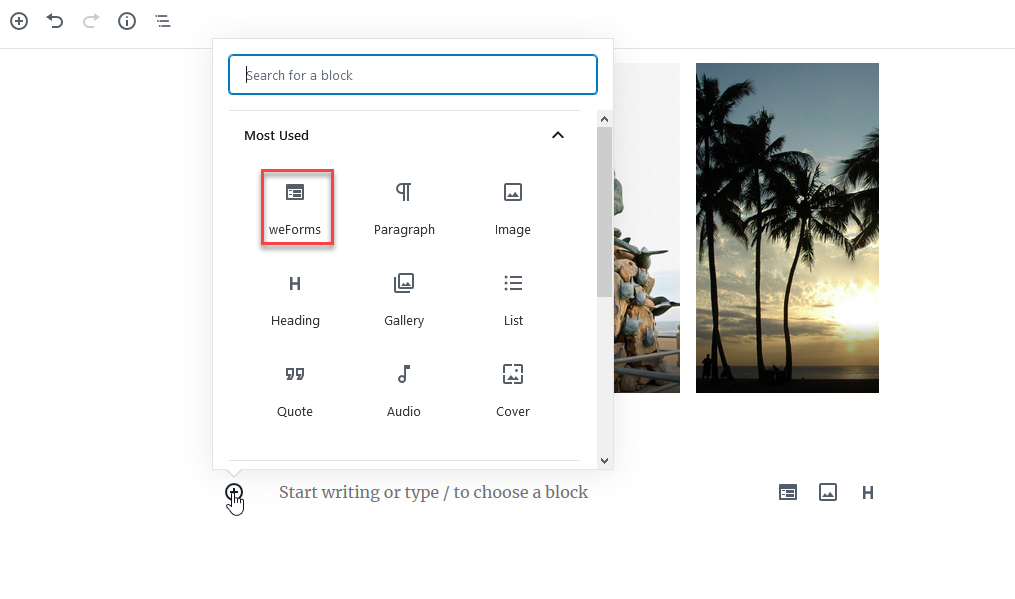The image is a horizontally rectangular screen capture, likely from a computer due to its shape and aspect ratio. In the top left corner of the frame, several icons are visible: a plus button, a back arrow, a forward arrow, an information icon, and a three-horizontal-bars menu icon. The focal point of the image is a pop-up window, which is square and contains a search field at the top labeled "Search for a block." Below this search field, there's a section titled "Most Used," featuring three columns of icons.

The first icon in the top-left corner, WeForms, is highlighted with a red border. The icons displayed, from top left to bottom right, are as follows: WeForms, Paragraph, Image, Heading, Gallery, List, Quote, Audio, and Cover. A scroll bar on the right side of the pop-up window suggests that additional icons are accessible by scrolling down.

To the right of the pop-up window, two images are partially visible. The first image is only partially seen with just its right edge shown. The second image, positioned further right, clearly depicts a scenic sunset framed by large palm trees, contributing a natural and serene backdrop to the interface elements in the foreground.